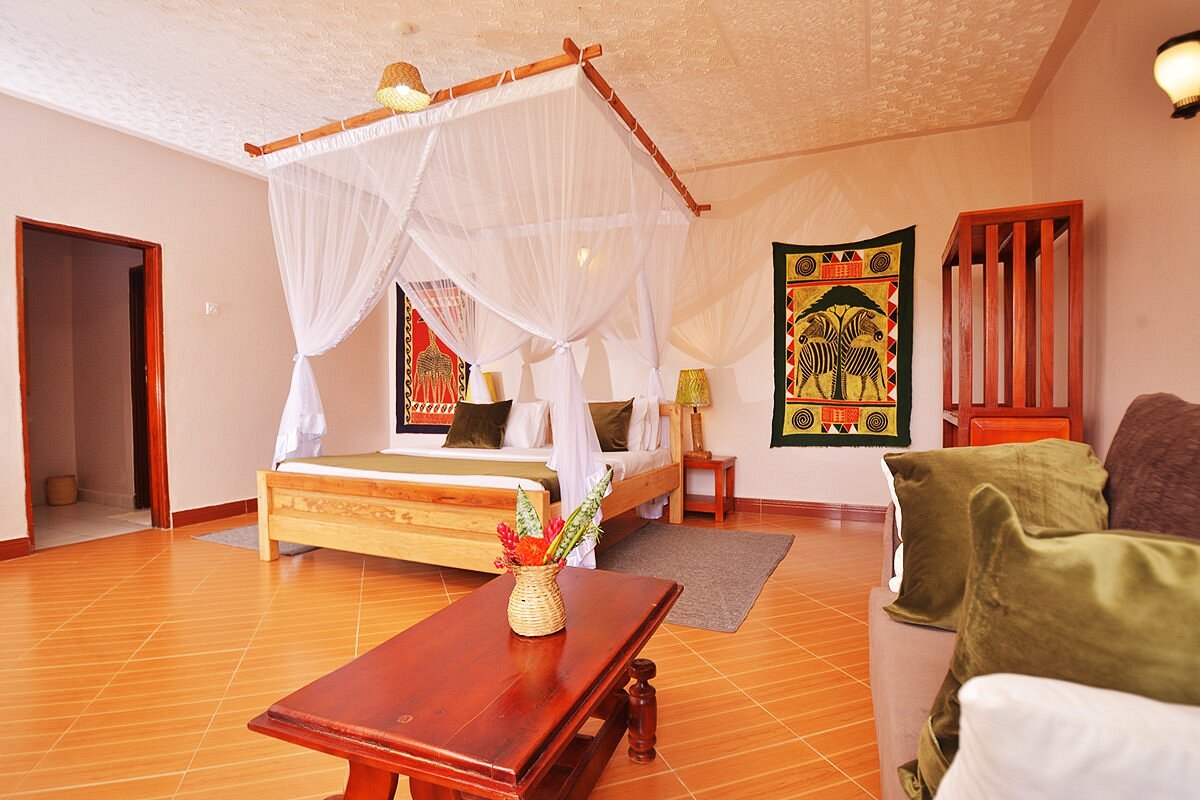This photograph showcases a modern, luxurious bedroom, possibly located in an exotic destination like an African or Asian hotel or resort. The room is adorned with a wooden-framed bed situated in the upper left corner, featuring crisp white sheets, a mix of white and brown pillows, a golden brown blanket, and a ceiling-mounted canopy designed for draping curtains or mosquito netting, albeit it appears unused.

The bedroom's floor is covered in an orange tile that resembles subway tiles with white grout, arranged to create a warm ambiance. On either side of the bed are long rectangular rugs. The walls are decorated with vibrant cloth wall hangings: on the left, a depiction of giraffes, and on the right, a tapestry illustrating zebras under a tree, adding to the room's eclectic and perhaps African-inspired decor.

To the right of the image, a tan couch with golden and green velvet throw pillows is complemented by a dark wood coffee table positioned in front. Additionally, a small brown table with a potted plant or flowers serves as a design accent in the foreground. Notably, the room lacks windows, focusing attention on its intricate and rich detailing.